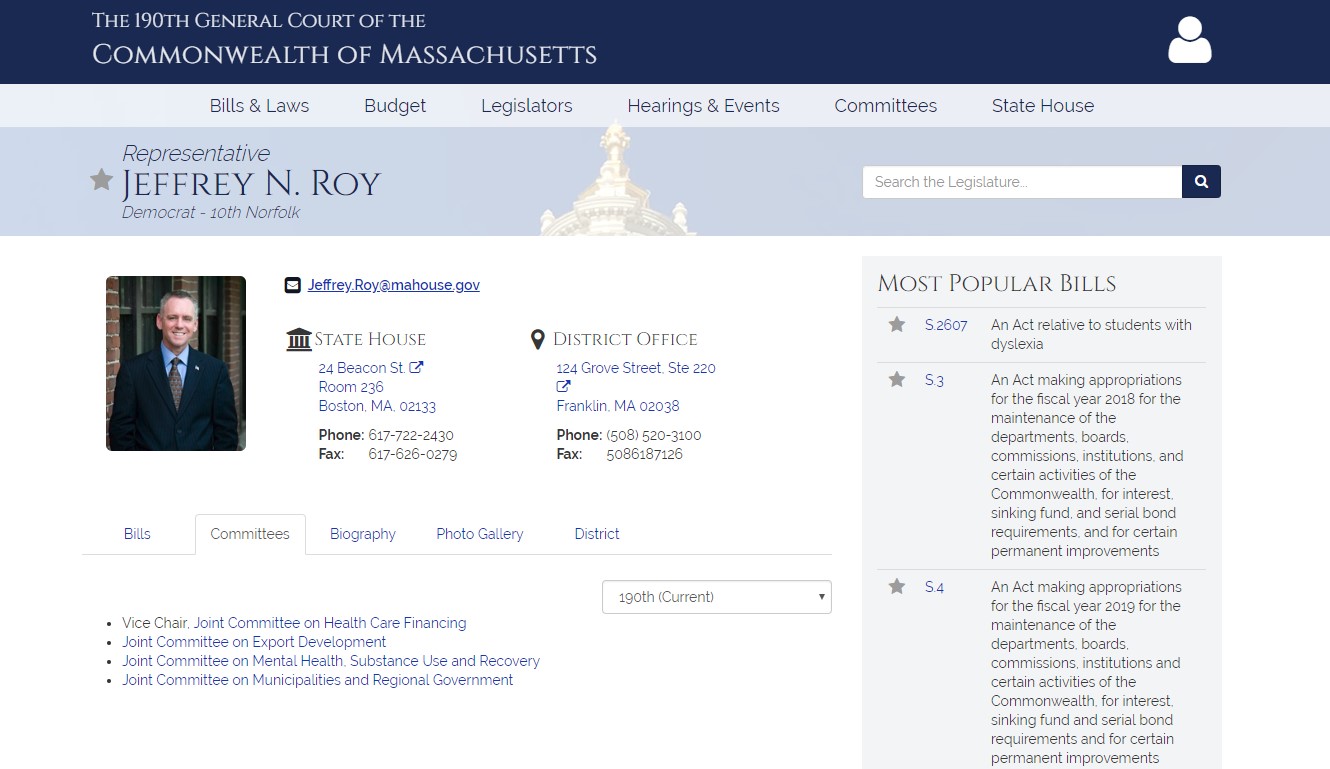A screenshot from the Commonwealth of Massachusetts website presents an in-depth bio page for a state politician. The webpage features a broad blue header at the top with the Commonwealth of Massachusetts prominently displayed on the left. On the right, there's a substantial profile icon depicting a stylized head and torso within a circle.

Beneath the header, a menu bar in small black lettering lists various categories: bills and laws, budget, legislators, hearings and events, committees, and statehouse. Further down, a large, faintly filtered header bar showcases the top of a capitol building with a blue overlay. To the left, the header identifies the politician as 'Representative Jeffrey N. Roy, Democrat, 20th Norfolk,' accompanied by a gray star icon. On the right, a small blue search icon box labeled 'Search the legislature' is prominently placed.

The section below this header prominently features Representative Roy’s picture on the left. To the right of his photo, details about his email, contact location, and district office information are provided. Beneath this section are five thumbnails categorizing information related to Representative Roy: Bills (sponsored), Committees, Biography, Photo Gallery, and District.

On the right side of the page, a large blue box at the top left reads 'Most Popular Bills,' followed by a vertical list enumerating the most significant bills.